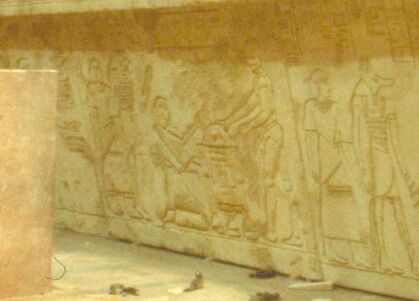The image appears to be a photograph of an ancient Egyptian wall relief or mural, depicting historical or mythological events. The wall itself has a yellowish tint, likely due to the age and materials used in its construction. The intricate carvings illustrate various figures and activities, unfolding a narrative of significant importance. On the right side of the image, there is a prominent figure with the head of a dog, likely representing Anubis, the ancient Egyptian god associated with mummification and the afterlife. Trailing behind this figure is another person who seems to be in motion, as if walking. The detailed craftsmanship of the artwork provides a glimpse into the sophisticated artistry and cultural richness of ancient Egypt.